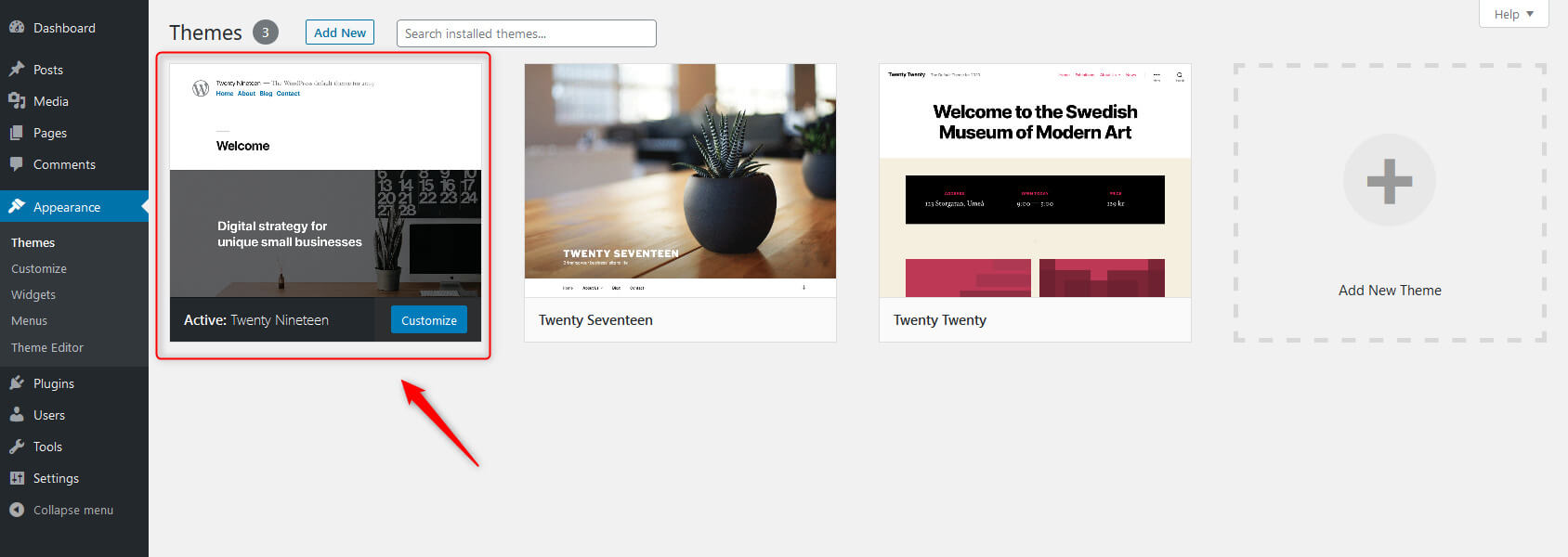This image is a long rectangular screenshot from a website, portraying a detailed web interface. On the far right side of the image, there's a tall, rectangular, gray menu panel featuring several clickable items. The menu items, displayed in gray text, are accompanied by small icons, making some of them hard to decipher.

At the top of the menu is the title "Dashboard," with an unrecognizable icon to its left. Below it is a push pin icon accompanying the label "Posts," followed by "Media" with another unclear icon. Next, "Pages" features two overlapping page icons, and "Comments" is marked by a speech bubble icon.

The menu progresses with a highlighted section in blue featuring white text: a paintbrush icon labeled "Appearance." Beneath "Appearance," there's a list of sub-options: 
- "Thomas" in white text
- "Customize," "Widgets," "Menus," and "Theme Editor" in slightly grayer boxes

Further down, the menu continues with:
- "Plugins" accompanied by a plug icon
- "Users" with a person icon
- "Tools" with a wrench icon
- "Settings" paired with a gear icon

Towards the bottom, there is a gray circle with a sideways-facing triangle labeled "Collapse menu" in black text.

To the right of this menu panel, the interface is dominated by a section with a faint gray background. At the top, above this section, it reads "Themes" in gray letters, accompanied by a gray circle with the number "3" in white. A blue-outlined square labeled "Add New" occupies the middle of this space, next to a white text box labeled "Search installed themes" in gray letters.

Below these controls are three and a half theme preview images:
1. The leftmost image has a red outline and a red arrow pointing to its upper left corner. Though the text is mostly unreadable, the top displays a white bar with the WordPress logo. Visible text includes "welcome" in black and "active 2019" alongside "customizing" in white letters inside a blue rectangular button. The bottom background of this image shows a gray wooden table with some small plants in white pots against a white wall.
   
2. The middle image features a blurry background of a room with windows. In the foreground, there's a wooden table and a circular bluish pot holding a small plant. White text towards the lower left reads "2017."

3. To the right, the next image has a white bar at the top with black text saying "Welcome to the Swedish Museum of Modern Art" and some unreadable small text above it. Below is a beige background, a long black bar with unreadable text, and two pinkish boxes. The bottom left corner reads "2020" in black letters. 

4. The half-image to the far right is an outline of a picture with a dotted border. Inside it, a gray circle with a plus sign indicates a placeholder labeled "Add New Theme" below.

At the upper right corner of this faint gray section is a clickable white box labeled "Help" with a downward-facing triangle.